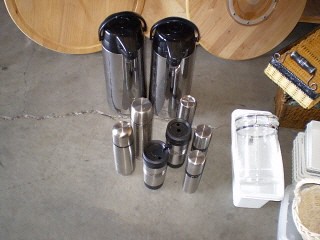The image depicts an arrangement of coffee supplies placed on a cement floor. At the front, there are small aluminium canisters and mugs, each with a black lid. Behind these are two larger metal coffee dispensers, also featuring black caps. To the right, there are additional items including white containers, a wicker basket resembling an Easter basket, and a basket that looks like it might be used for picnics. At the back of the scene, there are unfinished wooden tables laid on their sides. Two large circular wooden objects, which are possibly barrels, are also visible, adding an element of mystery. Enhancing the detailed assortment on the right side, a small table holds various items such as a yellow pack, a wrapped white object, and a few plates. This meticulously arranged setup combines functional coffee service elements with an eclectic mix of other supplies and background objects.